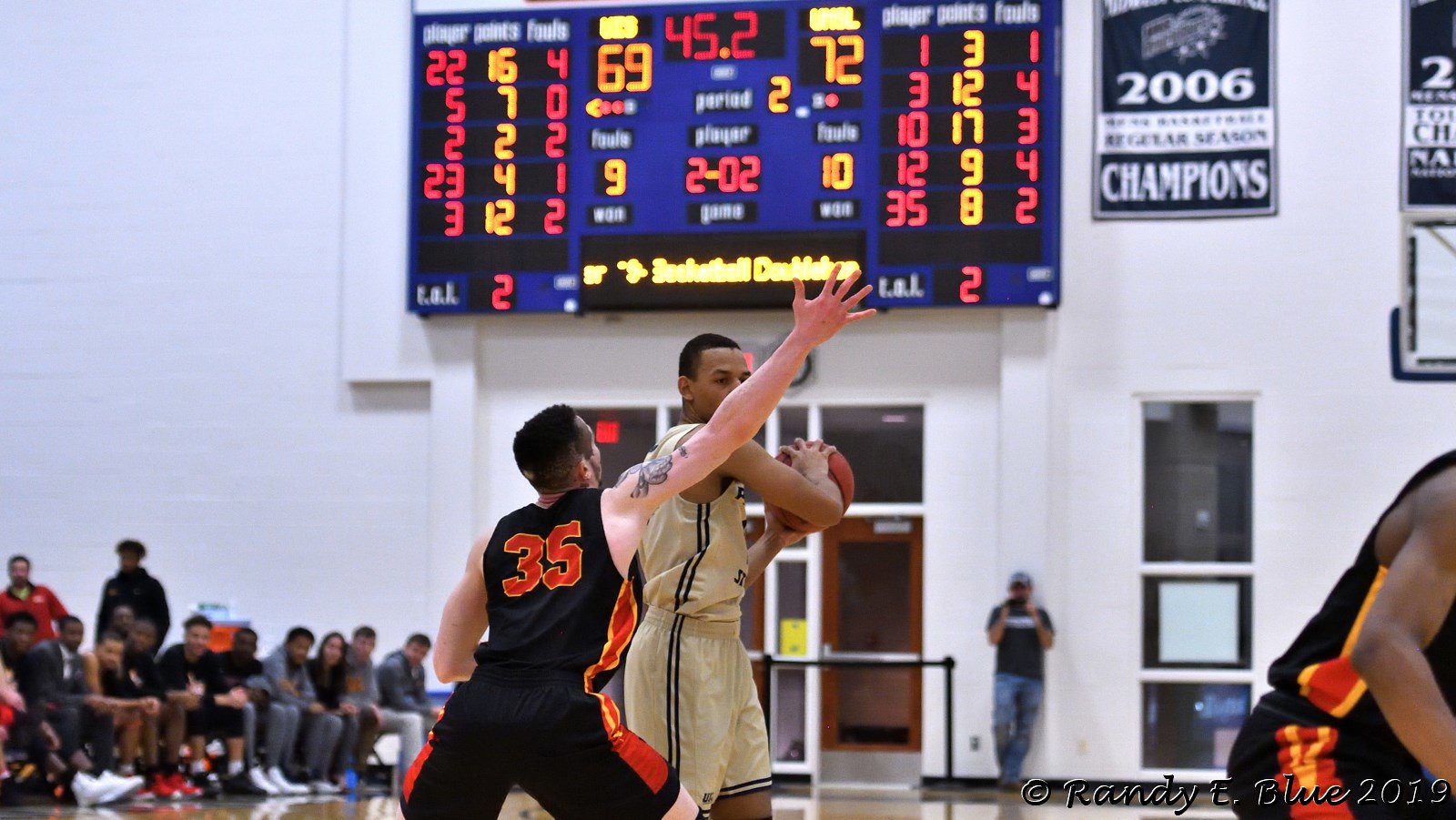This photograph captures an intense moment during a basketball game set in a gymnasium. At the center of the image are two primary players: the player on the left is wearing a black jersey with red accents and the number 35, contrasting with his white skin and black hair. He appears to be on the defense. The player on the right, who is Black with short black hair, is actively holding the ball and is dressed in a white jersey and shorts adorned with blue accents. Above the players, a blue scoreboard against a white gym wall displays a close score of 69-72. The gymnasium’s crowd is faintly visible in the background, albeit a bit blurred, adding to the game’s atmosphere. Notable above the scoreboard is a poster proclaiming "2006 The Champions." On the right side of the image, a couple of championship banners are visible, with the year 2006 being particularly prominent. The photograph is credited to Randy E. Blue, 2019, as indicated at the bottom right corner.